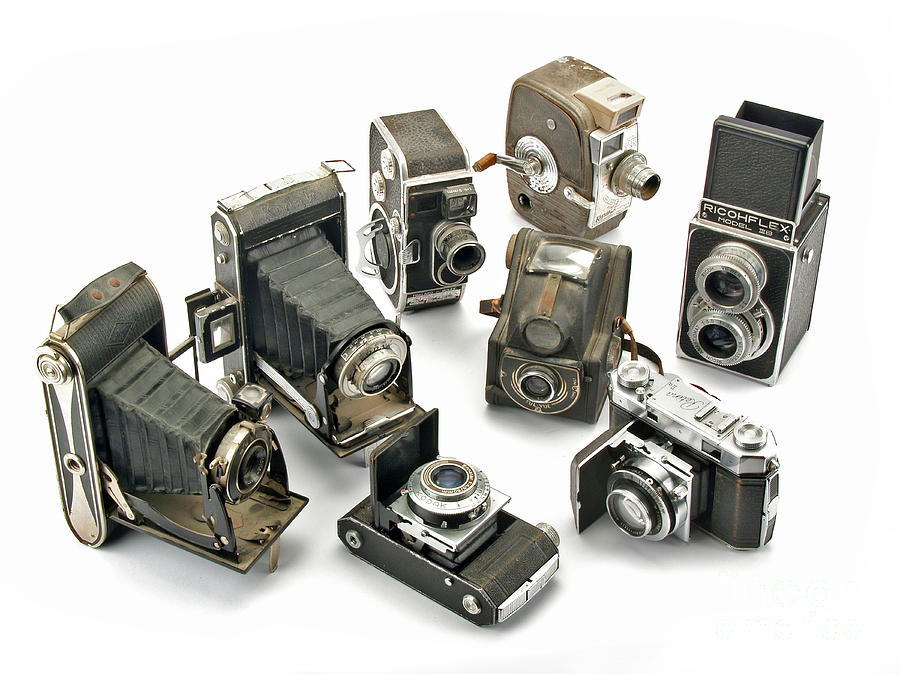This photograph showcases a collection of eight antique cameras, predominantly from the 1800s and early 1900s. The cameras are primarily black and silver, with some featuring leather components and evident brown dust, accentuating their age. Among them, two appear to be motion picture cameras, while the others are still cameras. Distinguishing characteristics include accordion-like extendable bellows, variously positioned lenses, and a mix of upright, angled, and laid-back orientations. Notably, the central camera, an extremely old faded brown model, faces the viewer directly. Several have features like knobs and handles, suggesting functional complexity. This image underscores the evolution of camera design, marking the transition from rudimentary forms to more advanced models.